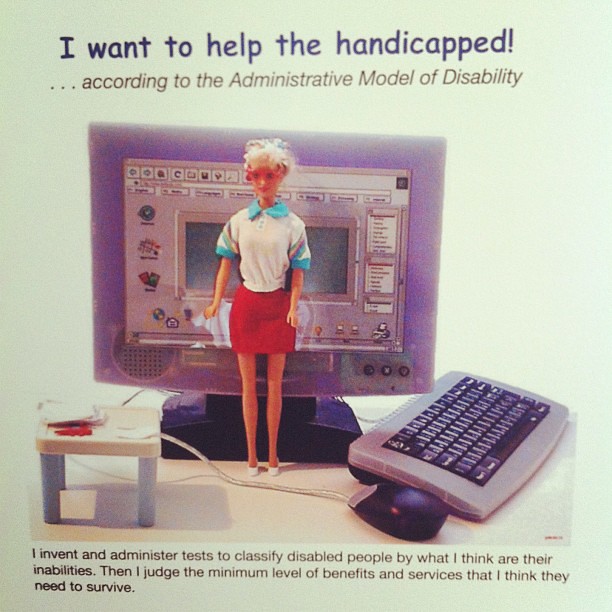The image depicts a Barbie doll with blonde hair, wearing pink glasses, a white shirt with blue short sleeves and collar, and a red skirt. She stands in front of a pretend computer monitor with an ambiguous screen, which has tool icons at the top, suggesting it may be for word processing. Near the Barbie on a plastic table are items including papers, a keyboard larger than the Barbie herself, and a mouse next to it. The background is green. At the top of the image, blue text reads, "I want to help the handicapped!" Below that, in black slanted script, it says, "according to the Administrative Model of Disability." Along the bottom, black text states, "I invent and administer tests to classify disabled people by what I think are their inabilities. Then I judge the minimum level of benefits and services that I think they need to survive." This seems to comment satirically on the way society classifies and assists handicapped individuals.